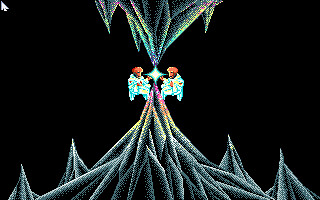The image features a black background contrasted by a central figure that resembles a frosted tree or an elaborate decoration. This main structure is adorned with intricate, shimmering details and extends upward with pointed tips. Directly above this element, a similar figure descends downward, mirroring the first with its own set of points. Connecting these two structures is a luminous star, positioned at their meeting point.

Flanking this star are two small, cartoonish figures. Each is dressed in white outfits accented with red headpieces and appears to be clinging to either side of the star, their eyes intently fixed on it. The whimsical nature of the figures adds a playful touch to the otherwise elegant scene. The overall composition, centered against the dark backdrop, creates a striking and surreal image, blending elements of nature and fantasy in a delicate balance.